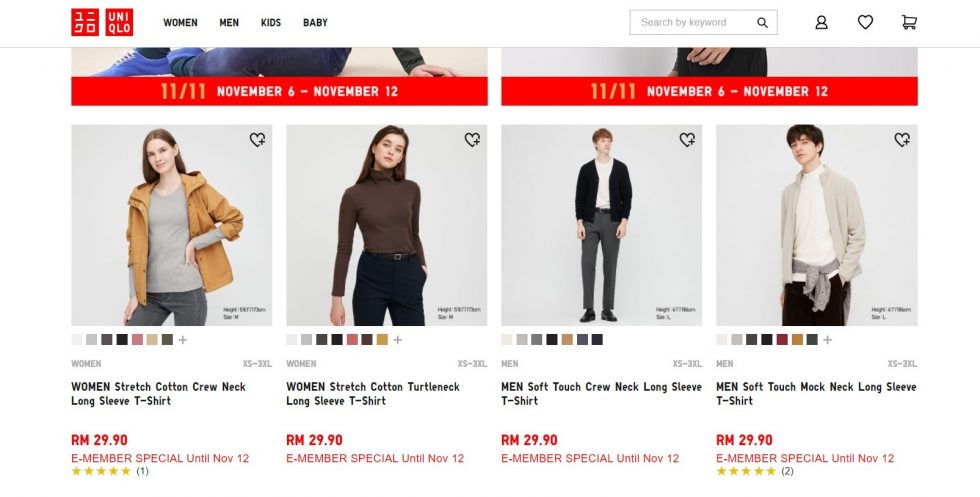This is a detailed caption for the given image:

---

The Uniqlo shopping page features a vibrant user interface showcasing Asian and English scripts in the top left corner against a striking red background, emphasizing the global reach of the brand. The header section is neatly organized with categories labeled "Women," "Men," "Kids," and "Babies." Adjacent to this, a gray-bordered search bar awaits keyword entries, highlighted by a magnifying glass icon for quick access. Additionally, the top right corner houses icons for user profile, favorites (heart icon), and shopping cart, each providing intuitive access to various user functions.

Beneath the header, two partial images are displayed with a consistent red banner featuring white text, promoting a special offer with the dates "11/11, November 6 through November 12." This section seamlessly transitions into four distinct clothing showcases, each spotlighting a featured item with vivid descriptions.

The first section presents an image of a woman with long hair modeling a tan parka-style coat over a gray shirt and blue jeans. The interface includes a heart-plus icon in the top right corner, suggesting an option to add to favorites, and additional text in the bottom right provides more details about the product. Color swatches below the image offer a variety of options including white, gray, brown, black, pink, tan, and olive, indicating the available colors for the showcased parka.

---